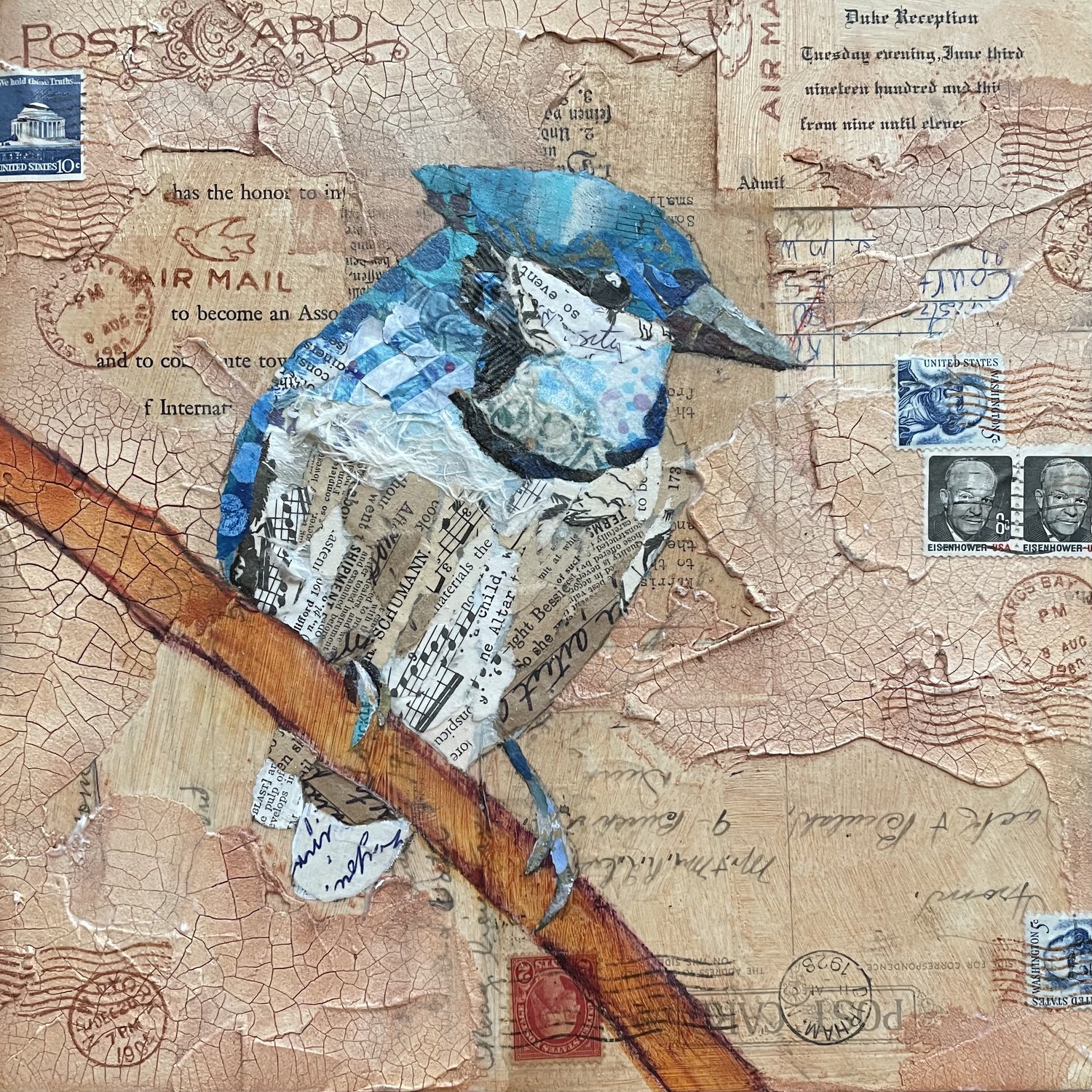The image showcases a detailed paper mache collage art piece depicting a blue jay perched on a branch. This intricate artwork utilizes various pieces of torn and clipped paper from a diverse array of sources, such as letters, envelopes, newspapers, postcards, and sheet music, which together form a larger cohesive image.

The foreground features a meticulously crafted bird, predominantly blue and grey, with its body composed of fragments from book pages and sheet music displaying musical notations. The bird's vivid blue head contrasts with the grey tones of its body, which utilizes text from newspapers and other printed materials.

The bird is perched on a brown-painted twig that diagonally stretches from the center bottom to the center left of the artwork. This twig comprises elements from a stamped envelope, with visible addresses, wrinkled paper, and parts of a postcard, enhancing its texture and depth.

The background is a textured collage of postcards and letters with visible stamps, including a five-cent United States stamp featuring George Washington, and two eight-cent Eisenhower stamps, along with a ten-cent airmail stamp placed in the top left corner. There are also postmarks and handwritten notes, some in an old-style script. Notably, the word "Postcard" is clearly visible in the top left corner. A beige, heavily textured paint overlay, which appears to be cracking, covers parts of these postcards, adding a vintage and weathered feel to the piece. Some legible text on the postcards includes a dated reception invitation from 1909 and other miscellaneous writings, contributing to the historical richness of the collage.